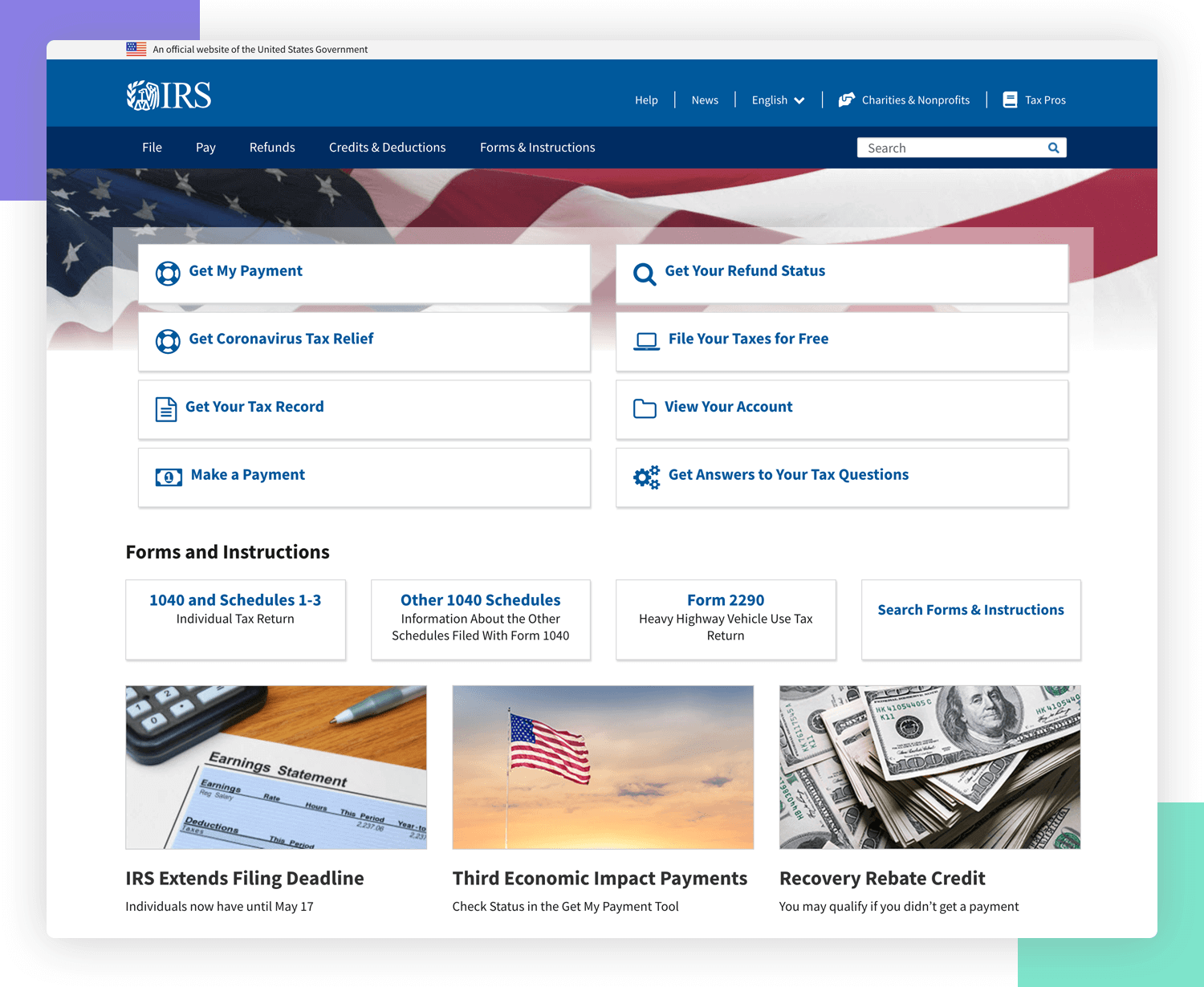The image shows a screenshot of the IRS website over a graphic background that includes a purple rectangle in the top left corner and a greenish-blue rectangle in the bottom right corner. The IRS website itself has a clean and structured layout with distinct sections. At the top, there is a white banner featuring the American flag, followed by a black text header, though the exact text is not legible. Beneath this is a long blue banner displaying the IRS logo and several navigation options, including a help section, and a few other features separated by vertical lines, including a drop-down menu and an icon labeled "Tax Plus."

Further down, there is a darker blue banner with navigation options in white text, reading: "File," "Pay," "Refunds," "Credits," "Forms," and an additional unreadable item. Towards the right side of this banner, a search bar is present with an image of the American flag in the background, gently billowing in the wind.

Below this, several interactive tiles are arranged parallel to each other, each with its own icon and label. They include:
- "Get My Payment" tile,
- "Get Coronavirus Tax Relief" tile,
- "Get Your Tax Record" tile,
- "Get Your Refund Status" tile,
- "File Your Taxes for Free" tile,
- "View Your Account" tile,
- "Get Answers to Tax Questions" tile.

These tiles are designed to facilitate easy navigation for users seeking specific IRS services.